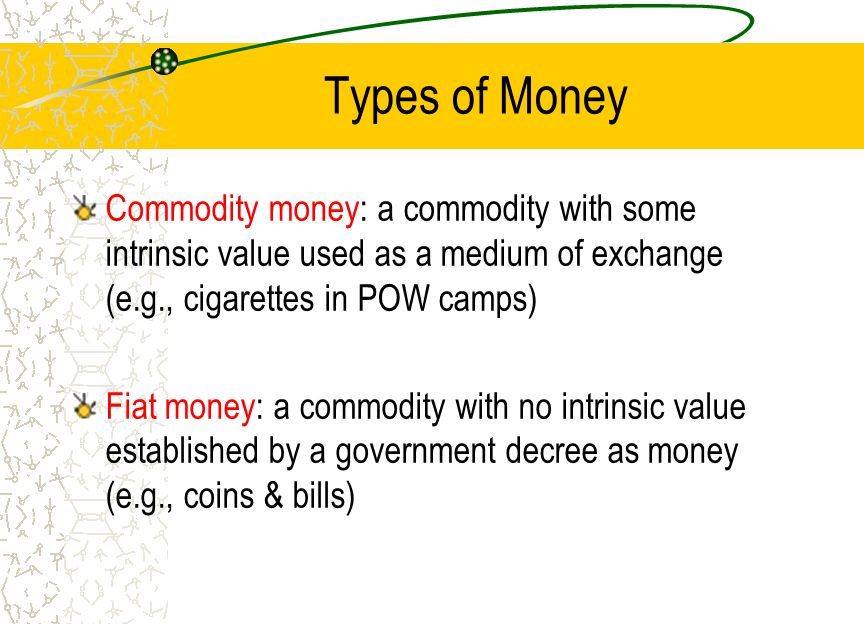The image is a slide or presentation page with a predominantly white background and a section on the left featuring an abstract gray pattern. At the top, a wide yellow banner spans the width of the image, overlaid with a subtle black swirl and white dots, with black text reading "Types of Money." A thin green line arches over this banner like a halo. Below the banner, two bullet points are listed vertically along the left side, each marked by a yellow symbol resembling a black spiky circle with a yellow center. 

The first bullet point, in red text, reads "Commodity Money: A commodity with some intrinsic value used as a medium of exchange (e.g., cigarettes in POW camps)." The second bullet point, also in red, states "Fiat Money: A commodity with no intrinsic value established by a government decree as money (e.g., coins and bills)." The majority of the text for each bullet point is in black font. 

The overall design is clean and typographic, presenting the information in a clear, infographic style.